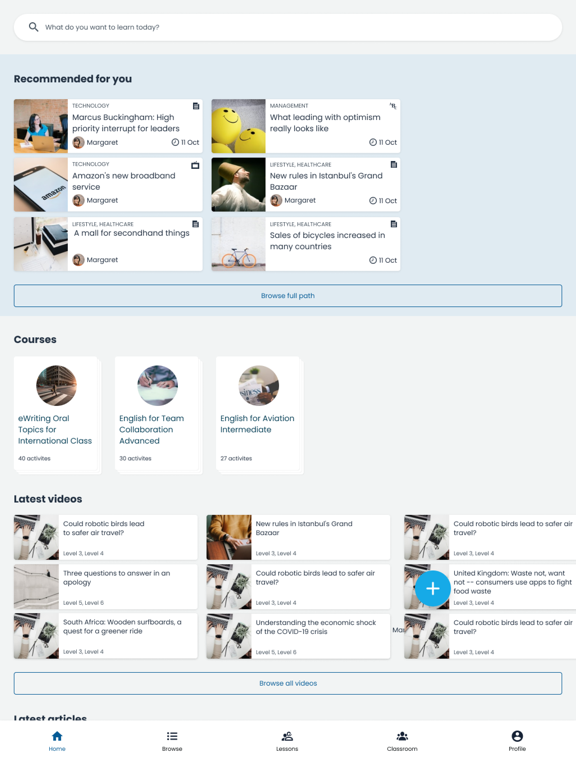This image showcases a well-organized online training platform with a sleek grayish-blue background. At the top of the webpage is a search bar, prompting users with the question, "What do you want to learn today?" Directly below, there is a bluish-gray box with the title "Recommended for you" at the top, featuring six white blocks arranged in a 3x2 grid. The first block highlights a course titled "Marcus Buckingham: High Priority Interrupt for Leaders."

Beneath this section, a "Browse Full Path" button invites users to explore further. Lower on the page, a "Courses" section showcases three available courses. At the very bottom, the "Latest Videos" section is divided into three columns, each containing three items, making a total of nine videos displayed. Additionally, on the right side of the image, there is a prominent blue circle with a white plus symbol, likely indicating an option to add or access more features.